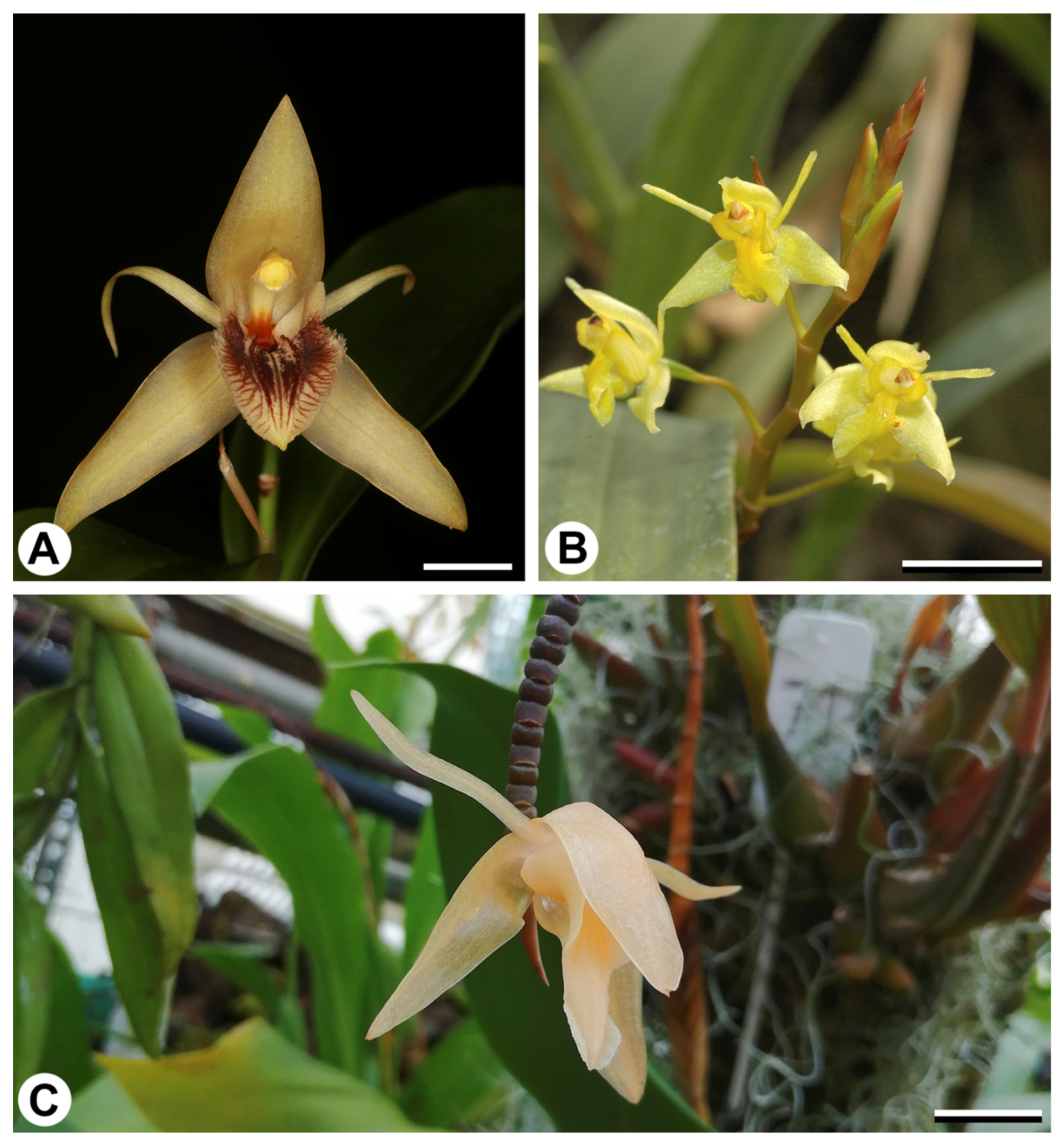The image is a composite of three photographs arranged in a grid, labeled A, B, and C. The top row contains two smaller images labeled A and B, while a larger image labeled C occupies the bottom row. All three photos depict the same type of star-shaped flower in varying stages of bloom and from different perspectives, showcasing detailed nuances in color and form.

In photo A, the flower is shown in a close-up view featuring a yellow star-shaped bloom with two tendrils extending from its center and a distinctive downward flap marked with crimson red streaks. The petals have a beige tint, possibly indicating the later stages of the flower's life. 

Photo B captures a more distant view, presenting three bright yellow flowers without the red streaks. These flowers appear to be in a fresher and more vibrant state, shown budding on a visible green stem. 

The larger photo C provides a different angle, depicting a single pale orange flower surrounded by green leaves. This flower appears healthier compared to A, but is slightly drooping, which might be due to its angle rather than its condition. The background includes green foliage, reinforcing the vibrant natural setting.

Overall, the series of images highlights the flower's lifecycle and diversity in appearance across different stages and angles.